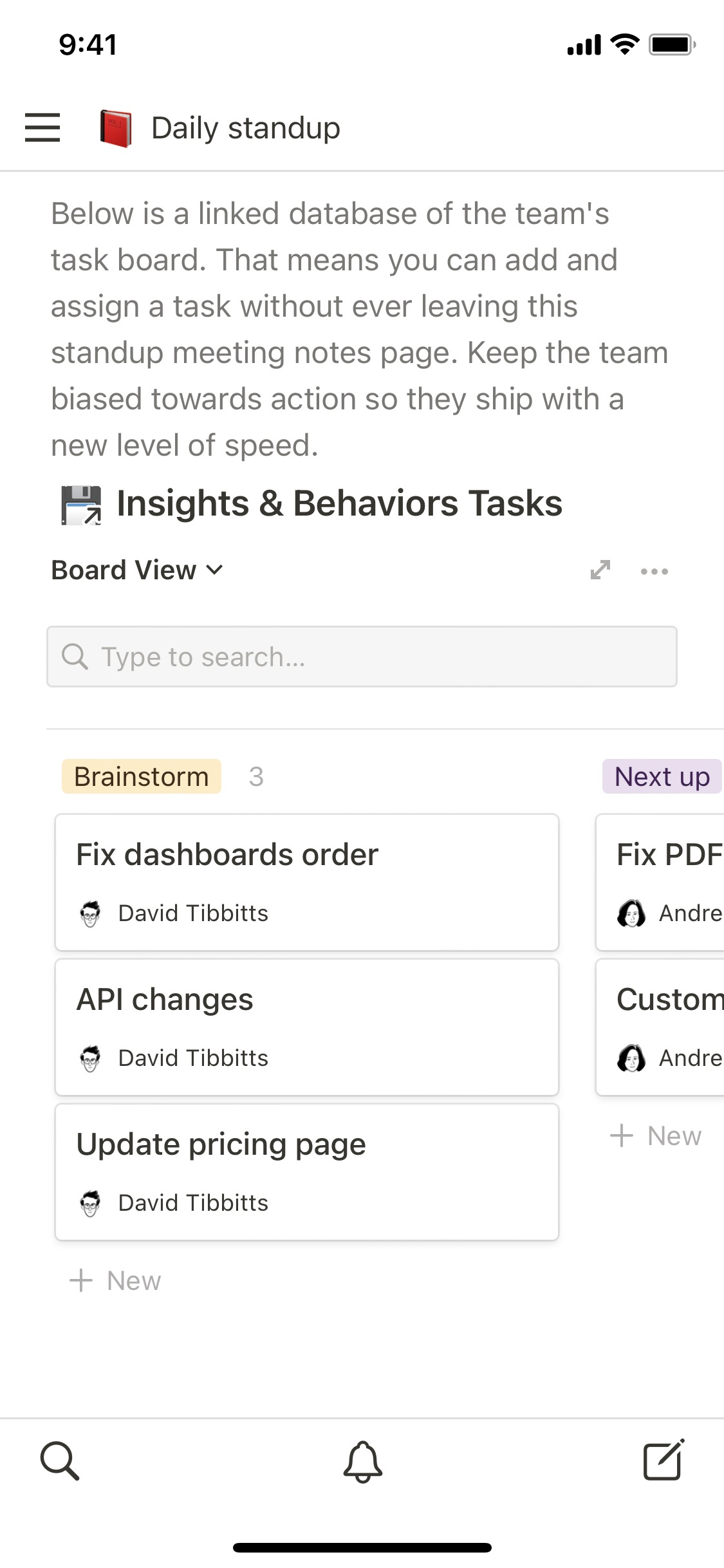The screenshot captured on a cell phone displays a portion of a productivity app interface. In the upper left-hand corner, the time is indicated as 9:41. The upper right-hand corner showcases several icons: cell phone reception, Wi-Fi, and battery status. Just below, on the left-hand side, the text "Daily Stand Up" is clearly marked, accompanied by an icon of a book. To the left of the book icon are three horizontal lines. Beneath this, a thin gray line serves as a divider. The next section contains the instructional text: "Below is a linked database of the Teams Task Board. That means you can add and assign a task without ever leaving the Stand Up Meeting Notes page. Keep the team biased towards actions so they ship with a new level of speed." Following this, there are labels for "Insights and Behavior Tasks" and "Board View." Directly below these labels is a search bar. The text "Brainstorm" is visible below the search bar, and to its right, the number three is displayed.